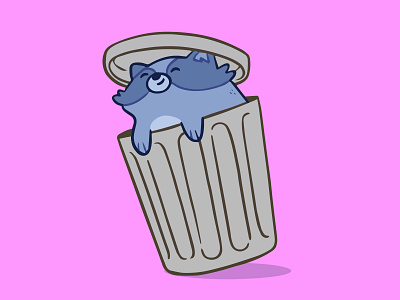This digital art drawing in a cartoon style features a raccoon peeking out of a slightly tilted, traditional metal trash can. The raccoon, adorned in shades of blue with dark blue patches around its eyes and ears, has a light blue muzzle and chest, while the rest of its body is a medium blue. The lid of the trash can rests humorously atop the raccoon's head. It is positioned partially out of the can, with little cartoon paws gripping the rim, and it appears to be looking up with closed eyes and a satisfied smile, as though it is enjoying the playful act of tipping the trash can over. The background of the image is a solid pink, and a shadow is cast beneath the lifted part of the trash can, adding depth to the whimsical scene.